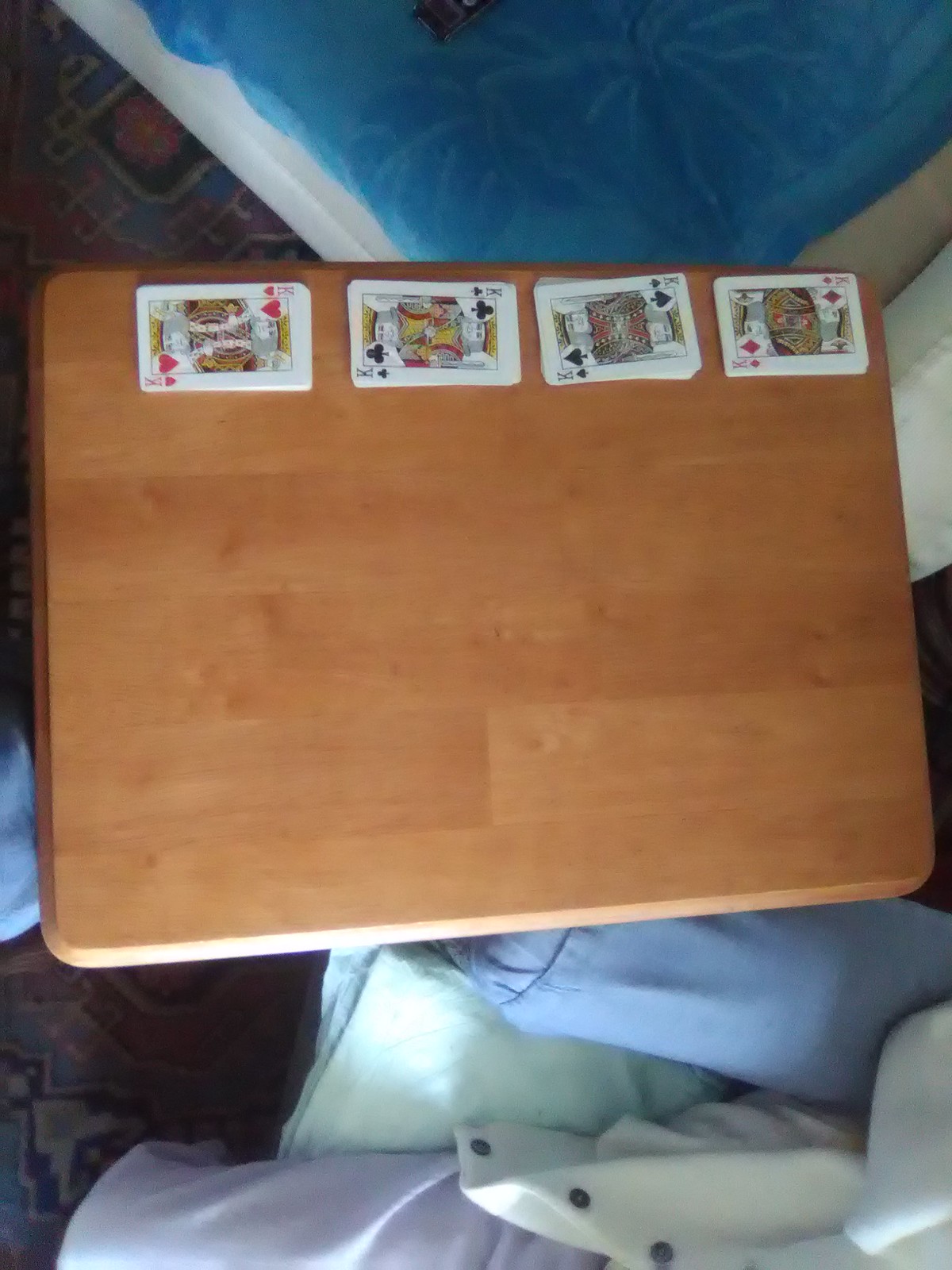This overhead photograph depicts a small, wood-topped table. At the bottom of the image, part of a blue overstuffed chair is visible, along with a woman wearing purple pants and a white button-up sweater. The table appears to be one that swings over a chair, suggesting a setting such as a hospital room. The top of the frame reveals what looks like a fiberglass walk-in shower, reinforcing the hospital room hypothesis. The chair also has additional padding for comfort.

On the tabletop, positioned away from the woman, a set of playing cards is methodically spread out. The face cards displayed are the King of Hearts, the King of Clubs, the King of Spades, and the King of Diamonds. These cards are arranged in four stacks along the edge of the table with the Kings facing up, though the rest of the cards in each stack remain hidden beneath. While it is logical to assume the cards are organized by suit, this detail cannot be confirmed from the image.